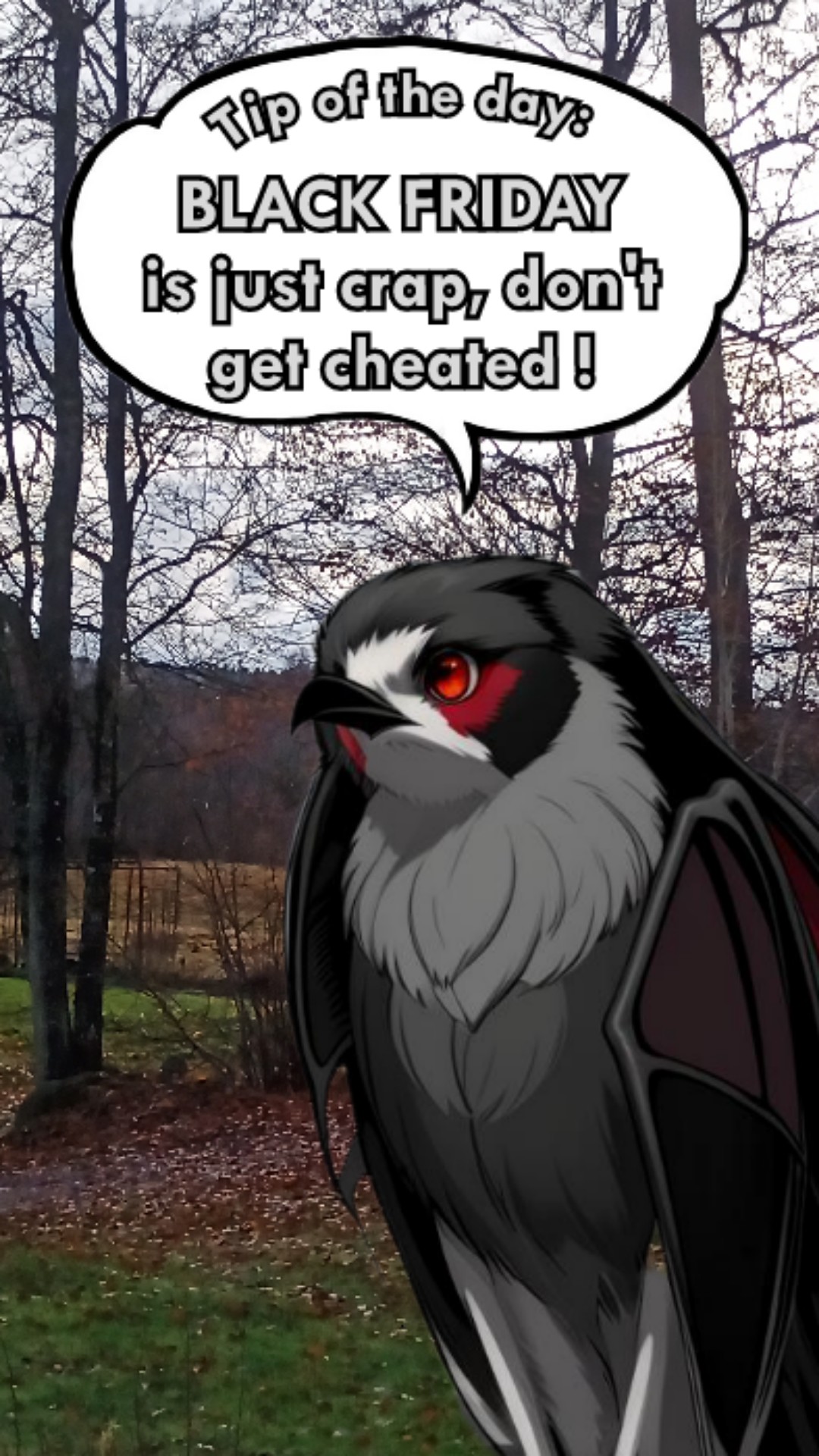The image features a striking contrast between a realistic fall landscape and a cartoony bird. In the background, a yard scene unravels with green grass strewn with brown leaves and a scattering of trees, whose branches are bare, suggesting late fall. Further in the distance, a field stretches towards a ridge of taller trees with some remaining foliage, capturing the serene essence of the countryside during daytime. Dominating the bottom right-hand quadrant of the picture is a graphic drawing of an owl (or possibly a bird of prey like a hawk or falcon). The bird is characterized by its predominantly gray feathers, red eyes, and a black beak, with additional color accents, including red around its eyes and white on its face, along with light gray neck scruff. Above the bird's head, a white word bubble with a black border contains a wry text in gray font: "Tip of the day: Black Friday is just crap, don't get cheated." This whimsical yet thoughtful image melds digital art with photography, making it an ideal piece for a card or social media post.